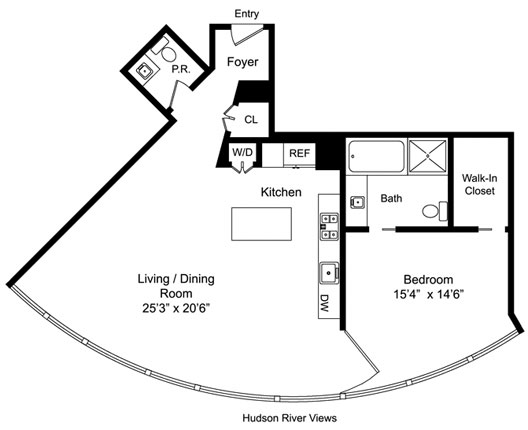Here is a cleaned-up and detailed caption for the provided image of the floor plan:

"This image illustrates the floor plan of a house. The bottom portion features a curved wall of windows labeled 'Hudson River Views' in black lettering, providing a scenic outlook. On the left side of the plan, a straight wall leads to an extended powder room, equipped with a toilet and a sink. Adjacent to this powder room is the foyer, which serves as the main entry point. Within the foyer, there is a closet with outward-opening doors.

Proceeding straight from the foyer, you enter a spacious living and dining room, measuring 25 feet 3 inches by 20 feet 6 inches. The kitchen, situated nearby, includes an island and features an L-shaped layout. It is equipped with a refrigerator, a cabinet for a washer and dryer, a cooktop, a sink, and a dishwasher. 

To the right of the kitchen counter, there is a large doorway that leads into a generously sized bedroom, which measures 15 feet 4 inches by 14 feet 6 inches. The bedroom includes a walk-in closet and an en suite bathroom. The bathroom is well-appointed with a tub, a shower, a toilet, and a sink."